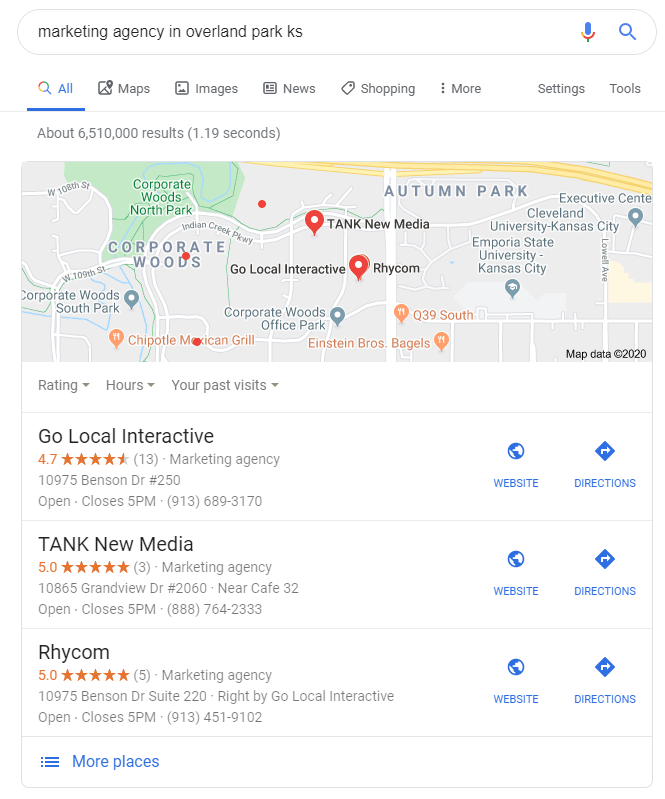The image displays a webpage featuring a search engine interface. At the very top, there's a search bar populated with the query "Marketing Agency in Overland Park, KS". Flanking the search bar on its right side is a microphone icon followed by a magnifying glass icon. Below the search bar, a horizontal row of tabs spans from left to right, including options labeled: All, Maps, Images, News, Shopping, More, Settings, and Tools.

Further down, the page indicates that there are "About 6,510,000 results (1.19 seconds)". Directly beneath this text, an image of a map is visible. Prominently displayed at the top-center of the map is the label "Autumn Park". In the bottom right corner, the map credits its data source with "Mapdata ©2020". Additionally, the map features a pinpointed label in the center, identifying a location named "Rightcom".